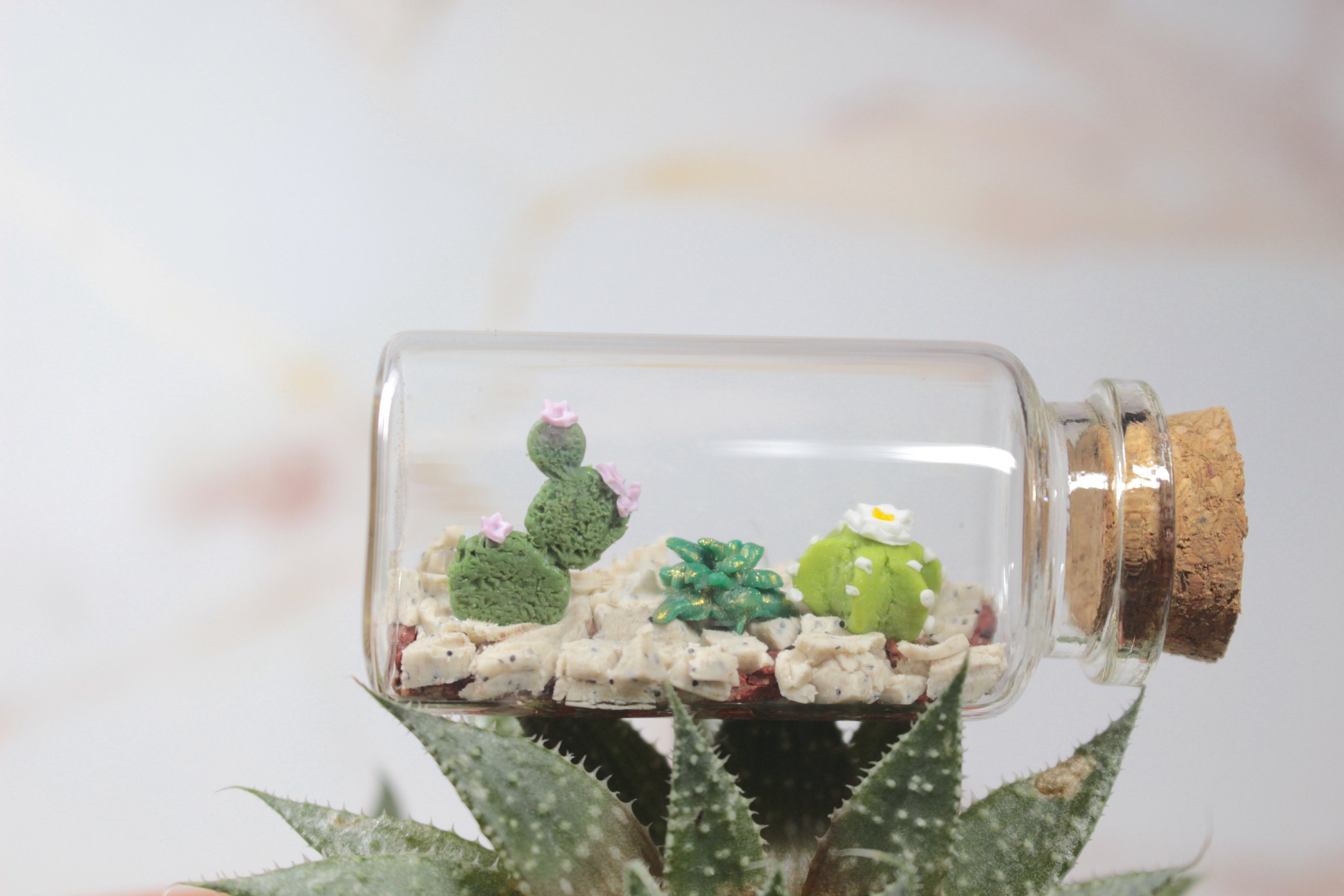This is a detailed close-up photograph of a small glass bottle, sealed with a cork, lying on its side atop a prickly, spiky green succulent plant. Inside the clear round bottle is an artistically crafted miniature garden scene, likely made from materials such as Play-Doh or ceramics. The base of this scene consists of small white rocks, upon which lie three distinct cacti. 

Starting from the right, there is a small round cactus decorated with pink flowers at the tops. Next, in the middle, there is a green cactus with white dots that appear to be either paint or ceramic, adorned with a white flower featuring a yellow center. Finally, a shorter leafy green cactus sits to the left with hints of gold paint accents.

The entire mini garden scene is meticulously designed, giving the impression of a desert within this tiny bottle. The bottle is balanced on the upward-pointing leaves of the succulent, which are sturdy enough to support it. The background is intentionally blurred, featuring soft hues of whitish gray, cream, and hints of pink and yellow, ensuring the main focus remains on the intricate details of the bottle and its contents.